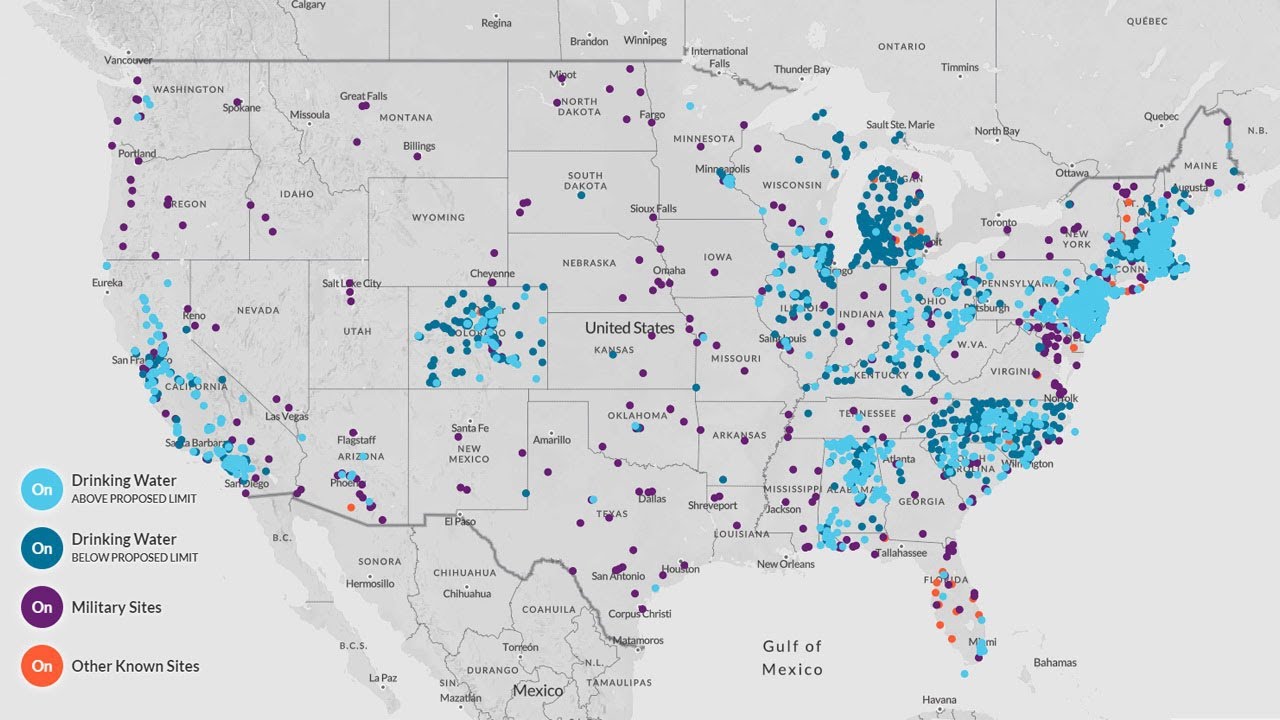This image is a detailed, digitally created map of the United States, highlighting various environmental and military topics using a color-coded legend. The map shows state boundaries, parts of surrounding countries (such as Quebec to the top right and Calgary to the top left, with Vancouver near Washington state), and major water bodies like the Gulf of Mexico.

The legend at the left side of the map explains the different colors of dots scattered across the states. Light blue dots indicate drinking water sources that exceed proposed limits, which are heavily concentrated in the Northeast, Carolinas, Colorado, and California. Dark blue dots represent drinking water sources that are below proposed limits, mostly found in Michigan and the Carolinas. Purple dots mark military sites and are sprinkled throughout the map. Orange dots designate other known sites, with significant clusters in Florida.

This comprehensive map is designed to visually represent important data regarding drinking water quality and site locations across the United States, making it an informative tool for understanding environmental status and distribution of military and other noteworthy sites.